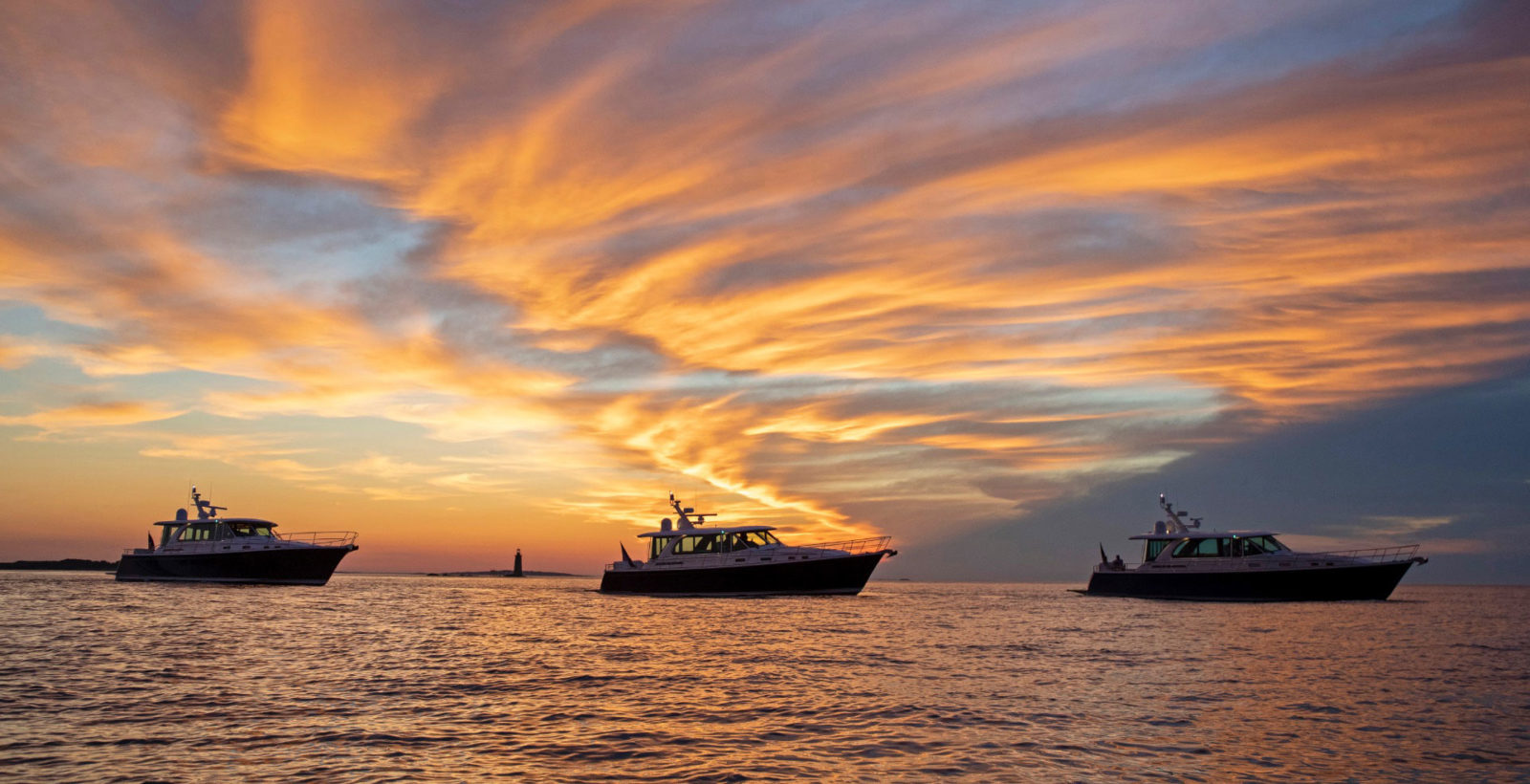In this up-close photograph taken during a dramatic sunset, three speedboats, all facing to the right, move in unison in a long convoy across the water. The predominant colors in the sky are vibrant hues of orange, pink, yellows, and blues, indicating the magic hour lighting of either dusk or late afternoon. Soft light still casts faint reflections on the water and the boats. The sky is filled with clouds highlighted by bright yellows fading into oranges, giving the scene a warm, ethereal atmosphere.

The boats are equidistant from each other, aligned left to right across the photo. The boat on the far right features a white stern trim on top and a darker underside, with handrails on its starboard side for safety. Moving left, the middle boat sits higher in the water, sporting a taller cabin, whereas the boat on the far left has a large, glassed-in cabin. Each boat has distinct features such as radar or wind vanes atop their cabins, distinguishing them from one another but sharing a similar overall structure.

In the distant background, just barely discernible between the second and third boats, there's a silhouette of a lighthouse or perhaps a long, narrow island-like structure that adds a focal point on the horizon. The scene's tranquility and warm tones evoke a sense of calm, poised at the transition between day and night.